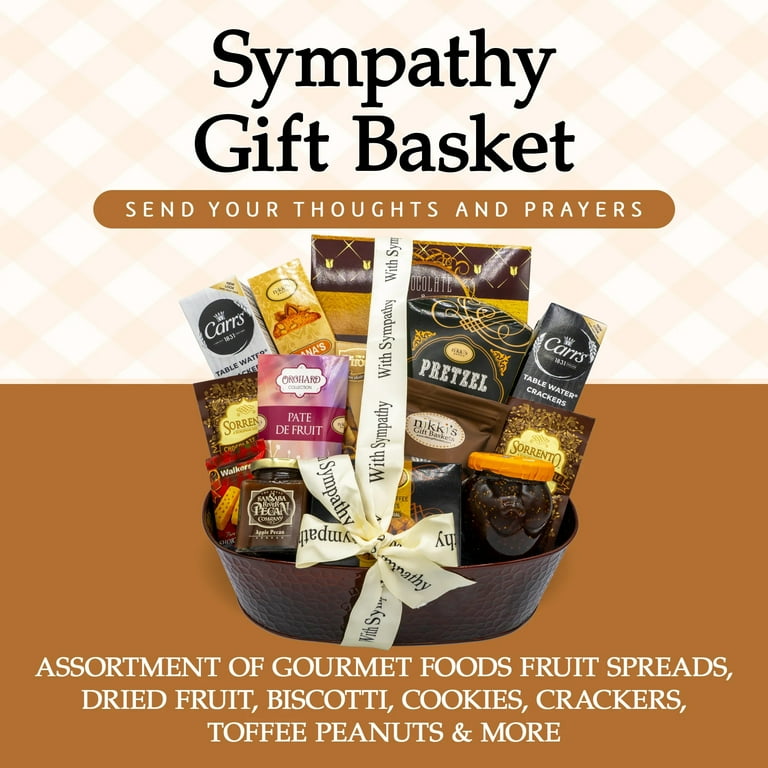This advertisement prominently features a sympathy gift basket under the headline "Sympathy Gift Basket" in black text. Below this, in capital white letters on a tan border, it reads "Send Your Thoughts and Prayers." The central image showcases a gift basket, specifically a brown metal oval container adorned with a cream-colored ribbon tied longitudinally with the repeated black-lettered message "With Sympathy." The basket is filled with a variety of gourmet items, including Carr's brand crackers, assorted pretzels, chocolates, teas, dried fruits, pistachios, pecans, and fruit spreads such as jelly. Visible treats also include Walker's shortbread, biscotti, cookies, and toffee peanuts, among other gourmet snacks. The bottom of the advertisement reiterates in white capital letters, "Assortment of Gourmet Foods, Fruits, Spreads, Dried Fruits, Biscotti, Cookies, Crackers, Toffee, Peanuts, and more." For more information, the ad provides a web address for additional details.